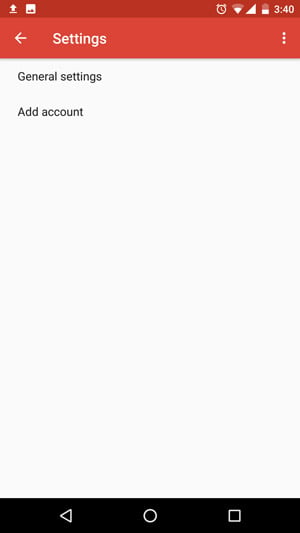The image depicts a new, sparsely populated webpage, likely captured from a smartphone or tablet. This is evidenced by the familiar bottom bezel which contains three icons: a left-pointing white arrow for navigation, a circle for collapsing the window, and a square for accessing open windows. 

At the top left, there's a prominent red bezel divided into two shades: a darker blood-red at the top, and a slightly lighter red below it. 

In the darker upper section of the bezel, several icons are visible: an up arrow with a line underneath signifying upload, a screenshot icon represented by a white box with silhouetted black mountains, a clock icon for setting an alarm, a Wi-Fi signal at two-thirds strength, a fully filled cell phone signal icon, and a battery icon showing approximately one-third charge. To the right, the time is displayed as 3:40.

The larger red section below contains a left-pointing white arrow labeled "Settings," and three ellipses positioned on the right side. Beneath this, in a light gray section, the text "General Settings" is displayed in black, with "Add Account" written below it.